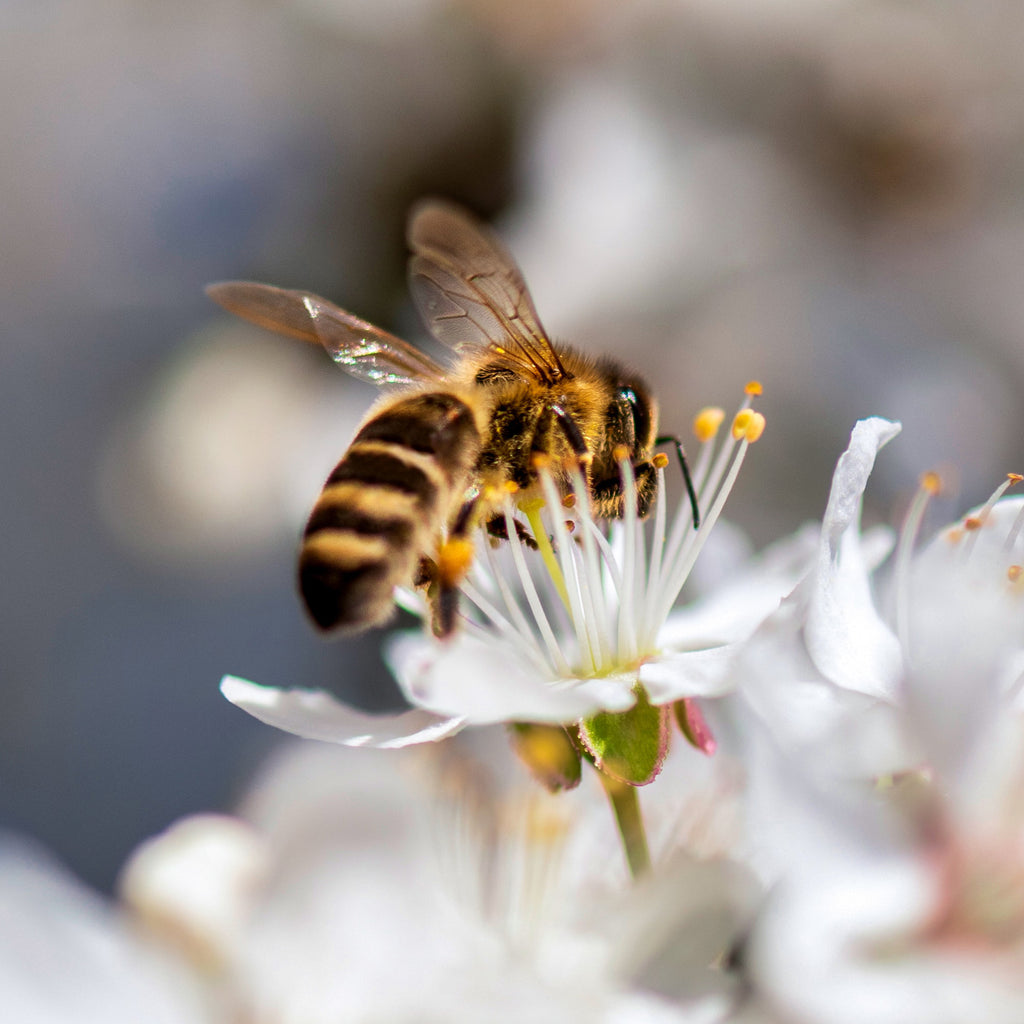In this detailed and close-up image, a bumblebee with the traditional yellow and black stripes is diligently pollinating a white flower, deeply immersed in its stamen. The bee's tail, striped in white and black, is prominently visible, pointing downward towards the bottom of the photo while its transparent wings extend outward. Surrounding the main flower are little round areas of green and red, and further below, there appears to be a cluster of additional white flowers, slightly blurred but identifiable at a lower level. The bee is centered in the image, showcasing its head and body with hyper-focused clarity. The background is predominantly gray and white, blurred to draw attention to the bee, though there are hints of brown and blue hues in certain areas. This natural scene emphasizes the bee's intricate role in pollination amidst a simple yet beautiful floral setting.